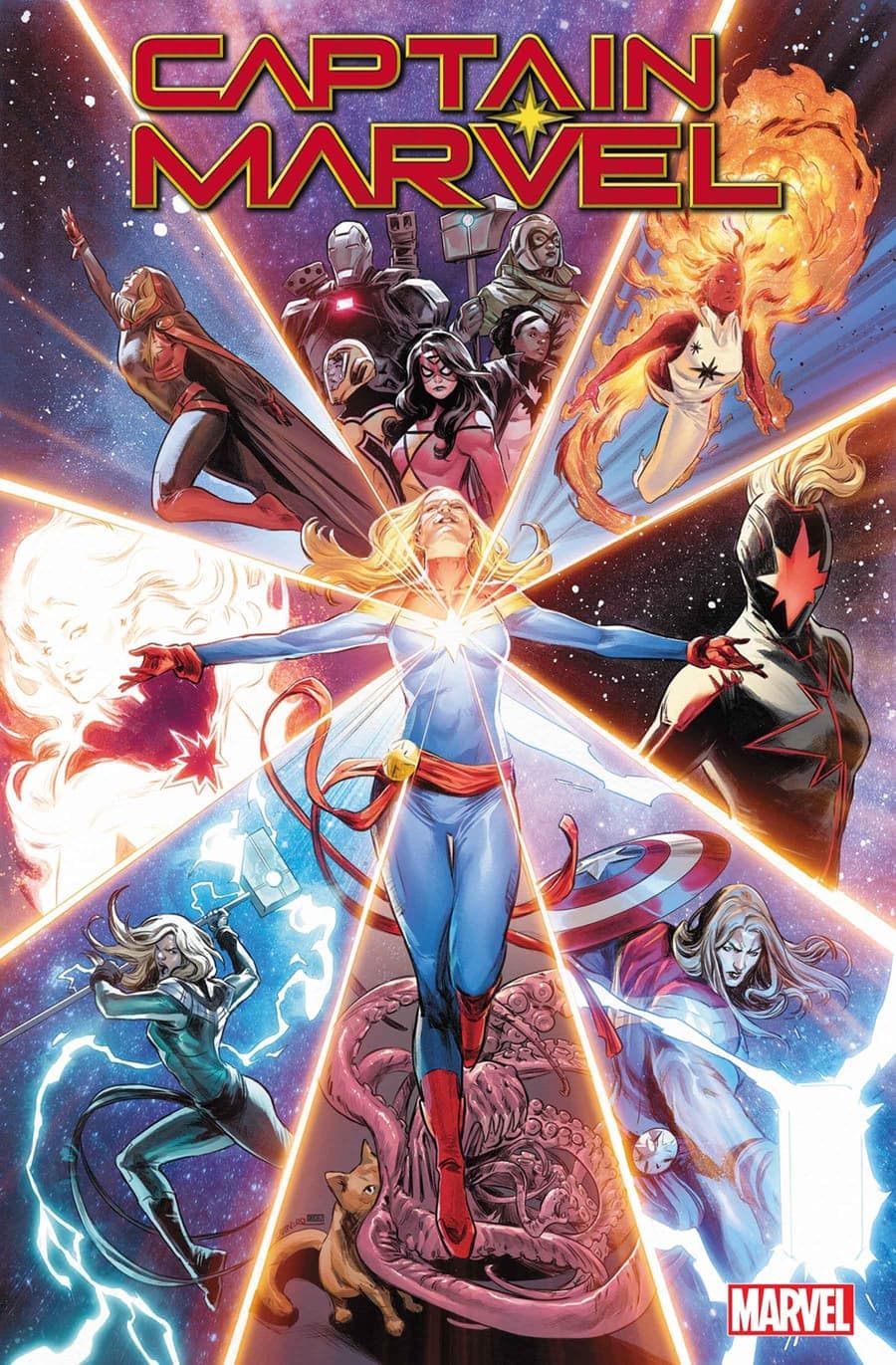This vibrant and highly detailed poster showcases Captain Marvel in a stunning array of colors including red, yellow, pink, white, and black. The title "Captain Marvel" is prominently displayed at the top in bold red letters with a yellow border, and a yellow star in the middle of it, making it stand out. At the bottom right corner, the Marvel logo is visible in white and red letters.

The central figure in the poster is Captain Marvel, depicted in a blue jumpsuit with a red sash, red boots, and red gloves. Light radiates from her chest emblem, emphasizing her powerful presence. Surrounding Captain Marvel are various other Marvel characters, separated by bright orange lines shaped like a star. Noteworthy among these characters is a figure resembling Wonder Woman in a blue jumpsuit with blonde hair, although this may be a misinterpretation commonly made by viewers. There are also elements like Thor's hammer and an alien-like figure with a cat next to it, adding to the captivating ensemble. The background includes stars, enhancing the cosmic theme. Overall, the poster is extremely colorful, lively, and detailed, effectively capturing the essence of the Marvel Universe.